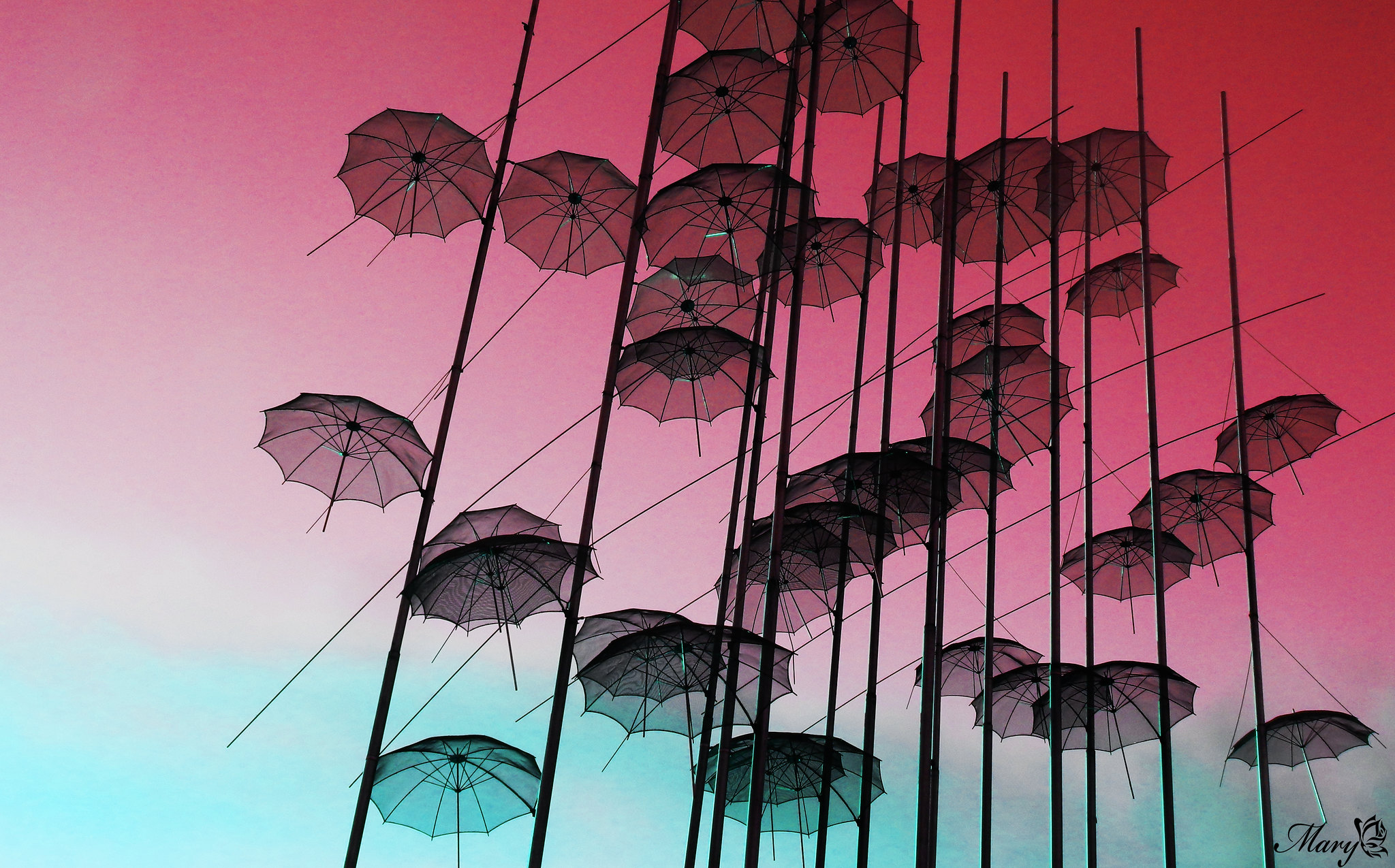The image is a drawing signed by Mary G. in cursive at the bottom right corner, accompanied by a butterfly sketch. It depicts a captivating art installation featuring approximately 20 translucent black umbrellas suspended in the air. These umbrellas are elegantly supported by a network of thin, black wire-like rods attached to larger, black poles that rise from the bottom of the scene. The background transitions from a light blue at the bottom to a gradient of pink, culminating in a deep dark pink in the top right corner. The semi-transparent nature of the umbrellas allows the underlying hues of blue and pink to subtly filter through, creating an ethereal and visually harmonious display.